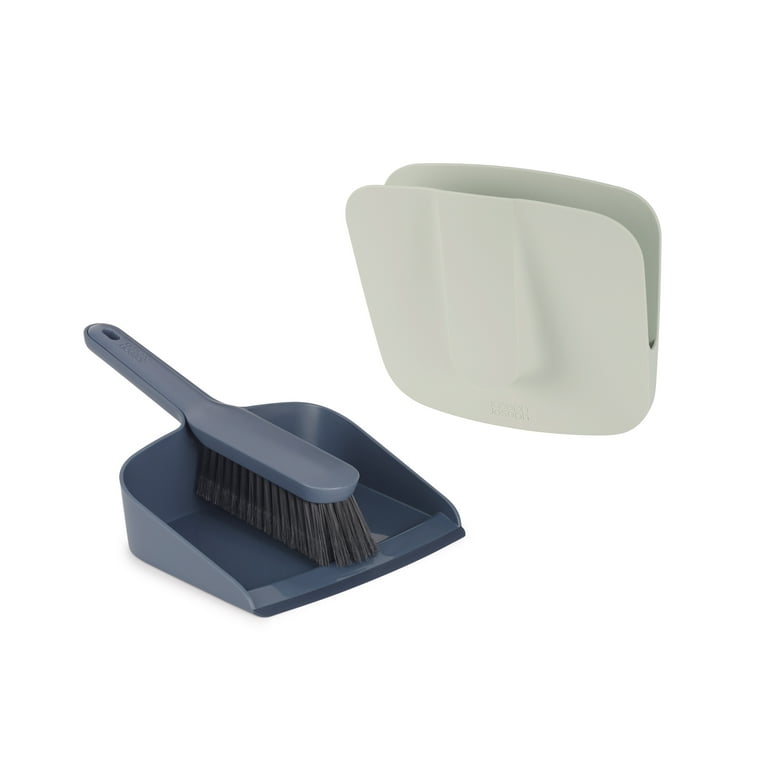The image depicts a cleaning set against a plain white background. Central to the image is a dark blue dustpan with an attached brush. The brush, which has black bristles, is designed to neatly nest into the handle of the dustpan, fitting snugly and forming a compact unit. To the right of the dustpan and brush set, there is a cream-colored, wall-mounted holder with an opening at the top, which features a noticeable indentation along its front edge. This holder appears to be designed either for storing the dustpan and brush set or as a small receptacle for collected debris. The image has no other objects or background details, suggesting it might be a stock photo intended for an online sale listing.